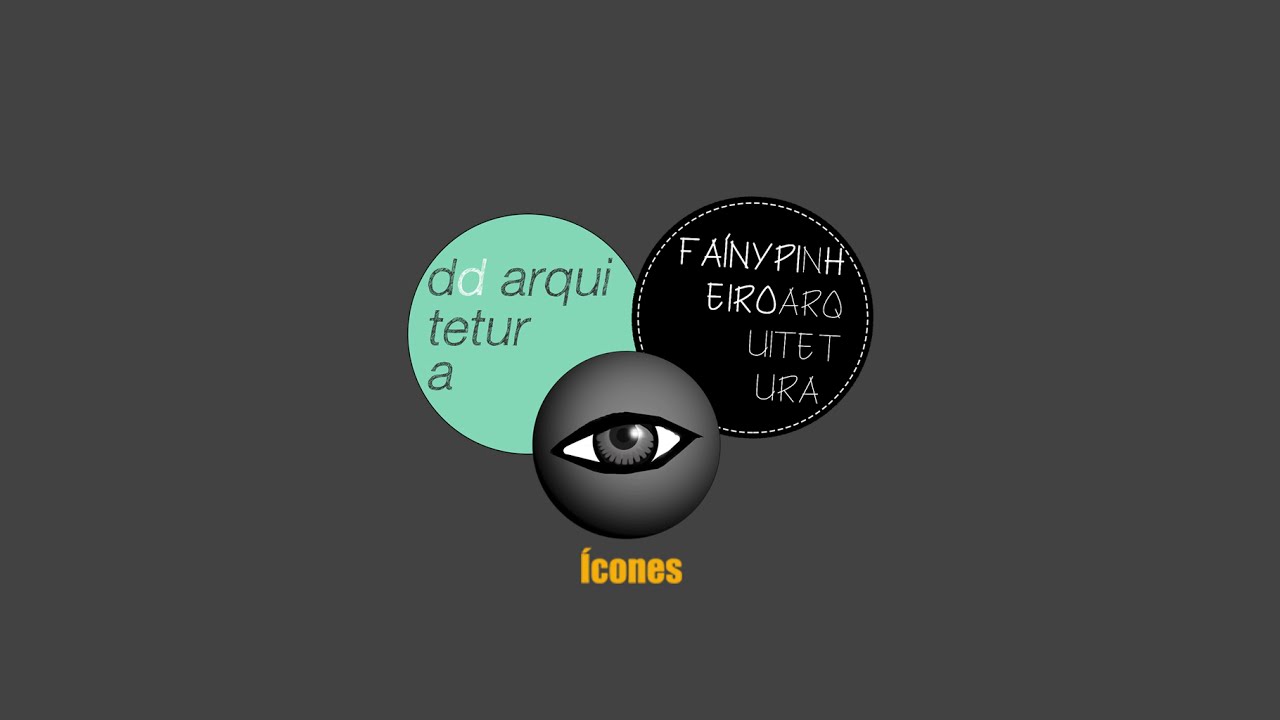The image appears to be a graphic frame, possibly from a PowerPoint presentation, with a solid dark gray background. In the center of this background are three overlapping circles: a large teal circle on the left, a large black circle on the right, and a smaller gray circle positioned in front and slightly below the two larger circles. The teal circle on the left features black lowercase text "d d a r q u i t e t u r a" with a single letter in white. The black circle on the right contains uppercase white font text "f a i n y p i n h e i r o a r q u i t e t u r a," appearing handwritten. The smaller gray circle in the front shows a stylized eye with a gray iris and darker shading around one side, giving it a spherical look. Below these circles, on the dark gray background, the word "I c o n e s" is written in a lowercase yellow font, with an accent over the letter "I".